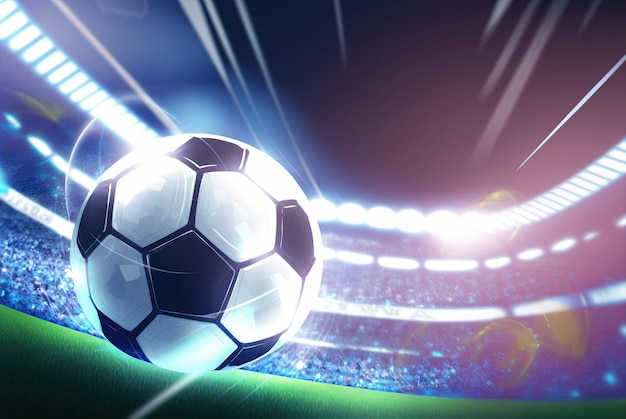The image depicts a digitally created, cartoon-like scene of a traditional black and white soccer ball in motion, prominently displayed on the bottom left side of the frame. The soccer ball, composed of pentagon and hexagon panels in a classic design, appears to be flying or rolling, indicated by white motion lines and swooshes surrounding it. The scene unfolds within a large, brightly lit soccer stadium at night, where numerous dots substitute for the crowd, suggesting a full house. The vibrant stadium lights illuminate the upper part of the image, enhancing the night setting while leaving the sky largely indiscernible. The green turf stretches diagonally across the bottom of the frame, showcasing a slight angle and some orange discoloration in the bottom right, mimicking a blur effect. The overall atmosphere conveys a sense of dynamic movement, with the ball appearing shiny and almost reflective, suggesting it might be part of a poster or video game screenshot.